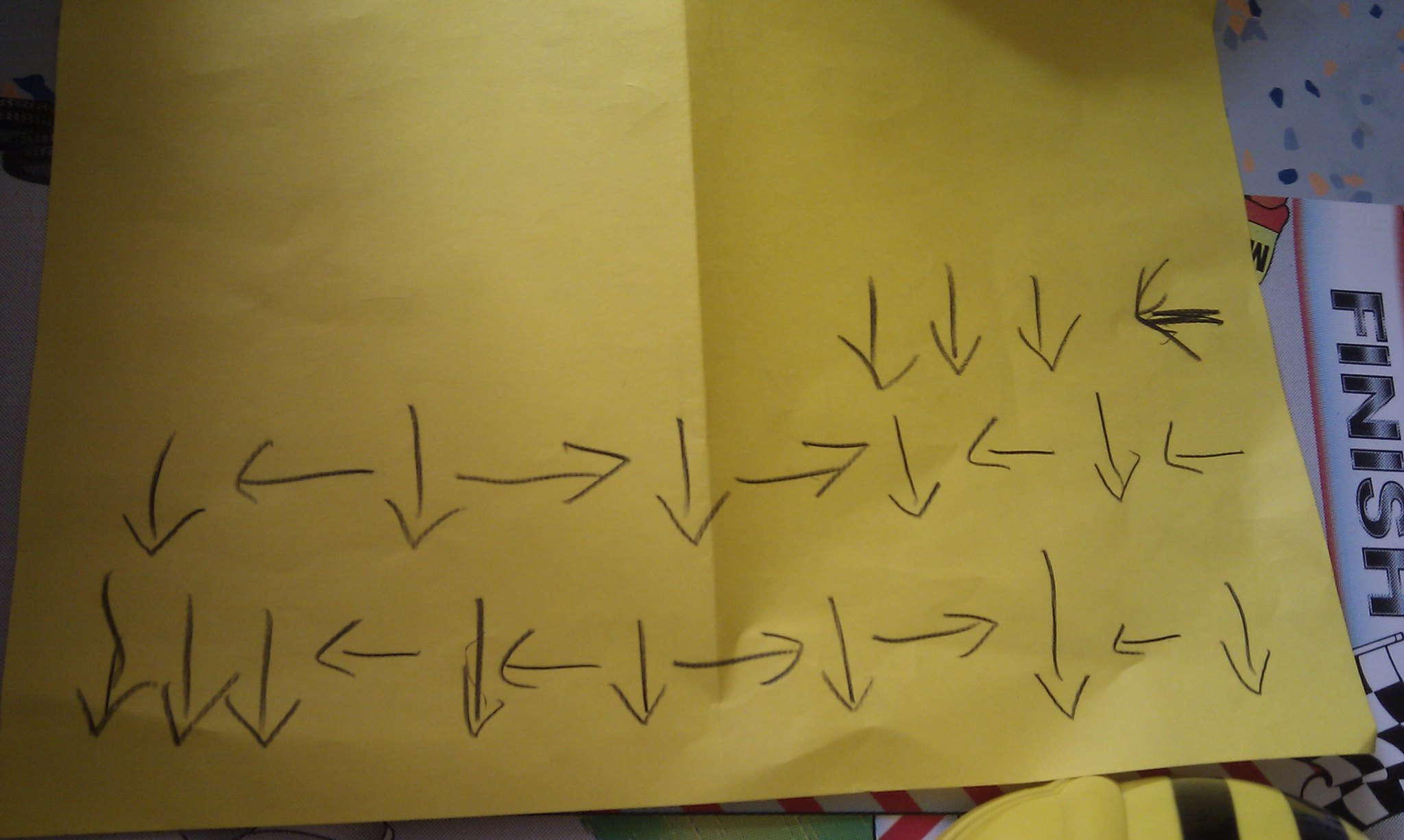This photograph features a large sheet of white construction paper positioned on a table that is surrounded by various decorating items scattered on the floor. On the construction paper, numerous arrows are drawn using either a black crayon or marker. The arrows are oriented in various directions: some pointing left, some pointing right, and some pointing downwards, but none are directed upwards. The arrows appear to be arranged in three disorganized rows with no discernible pattern. The scene suggests a creative or instructional project amidst an untidy workspace.